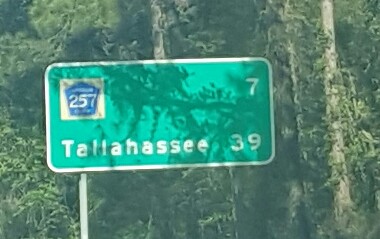In this serene outdoor scene, a lush forest of pine trees dominates the background, creating a tranquil natural setting with no animals or people present. Sunlight gracefully filters through the foliage, casting a gentle glow. In the foreground, a prominent green highway sign with a white trim stands out. The sign indicates the distance to Highway 257, which is 7 miles away, and further indicates that Tallahassee is 39 miles ahead. The sign's light green surface is partially shaded by the silhouettes of nearby trees, adding a dynamic contrast to its appearance.